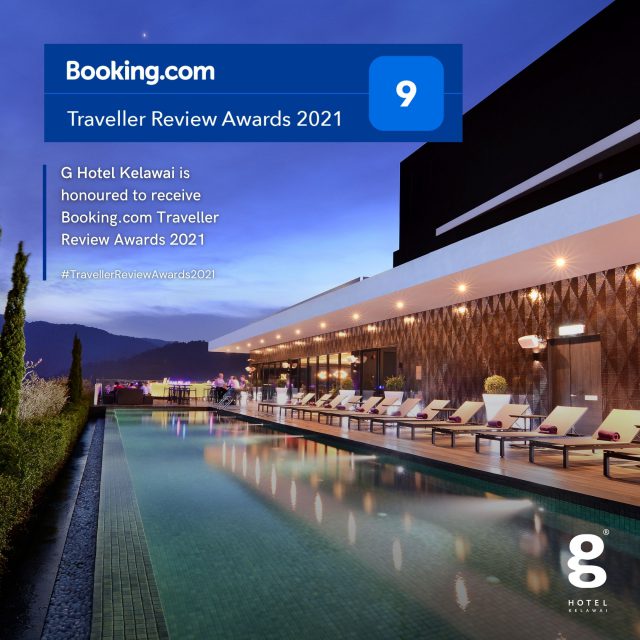This image appears to be an advertisement for a luxurious resort featured on Booking.com, showcasing a serene, modern, and elegant poolside setting at the G-Hotel Kelowai, which proudly displays its accolades.

The background captures a picturesque view of this sophisticated resort during the evening. The scene is dominated by an opulent outdoor area adorned with numerous meticulously arranged poolside lounge chairs, each equipped with a neatly rolled towel. The lounge area lines a long, rectangular pool filled with crystal-clear water, softly illuminated by underwater lights, evoking a tranquil and inviting ambiance.

On the left-hand side of the setting, lush plants form a natural border, adding a touch of verdant beauty to the scene. The far end of the pool reveals a breathtaking mountainous backdrop, silhouetted against a darkening evening sky, painted in twilight hues. The building itself is lit up, hinting at the warm, welcoming atmosphere of the interior.

For a touch of human presence, the distant left side of the image showcases a seated group, subtly adding life to the tranquil setting. 

Overlaying the top left of the image is the recognizable Booking.com branding within a dark blue rectangle. This contains the site's name in bold white letters, a light blue line beneath, and a small square with the number '9' in white encased in the same dark blue, symbolizing a high rating. Below, the text proclaims "Traveler Review Awards 2021."

Additionally, placed on top of the image in white text, the advertisement proudly announces, "G-Hotel Kelowai is honored to receive Booking.com Traveler Review Awards 2021," accompanied by a vertical blue line to the left for design enhancement. The bottom right corner of the ad is adorned with a stylish white lowercase 'g', the logo for G-Hotel Kelowai, emphasizing the hotel's brand identity.

This comprehensive display not only highlights the beauty and elegance of the G-Hotel Kelowai but also its esteemed recognition, making it a compelling visual piece for potential travelers.